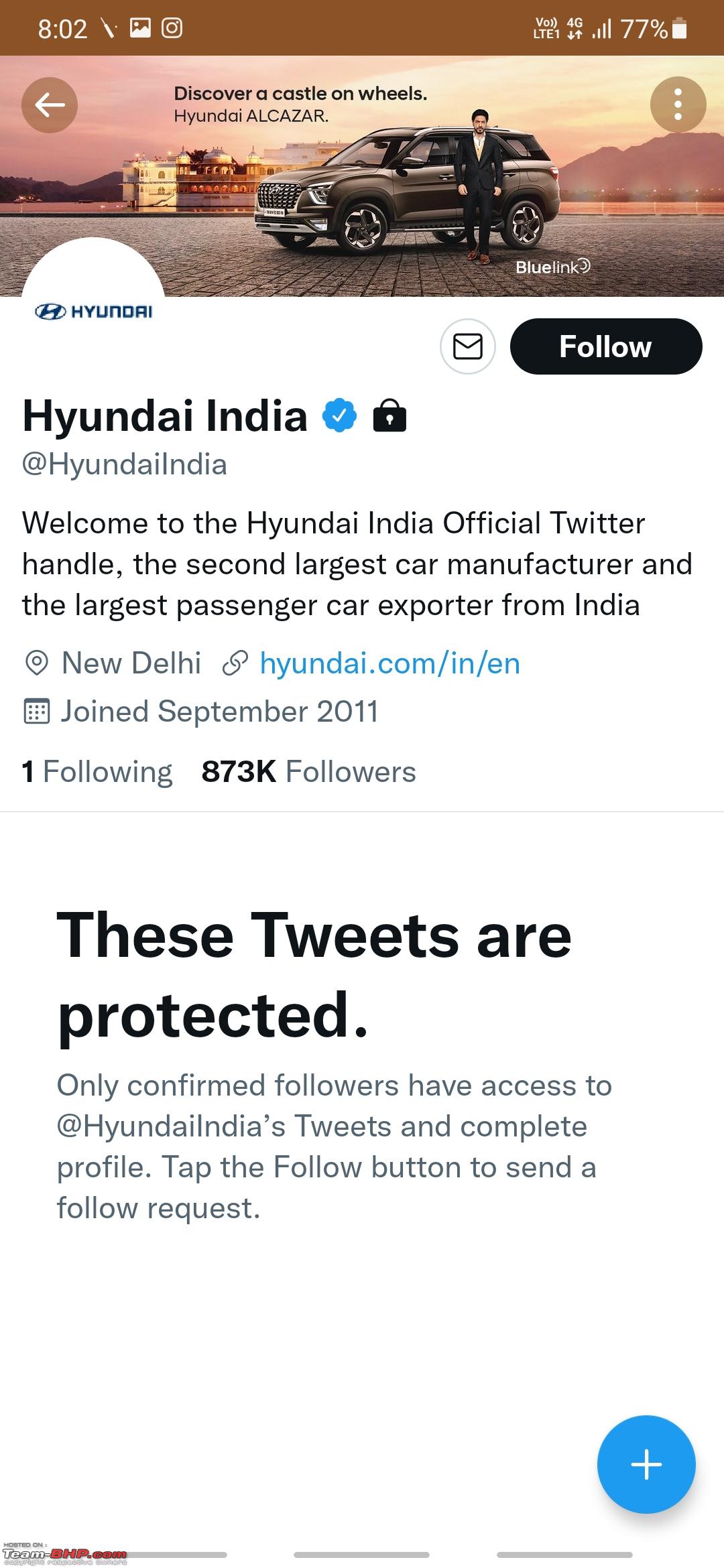The smartphone screen displays the official Hyundai India Twitter (X) page. At the top, the screen's status bar shows a dark brown banner with the time as 8:02 and a battery life of 77%, alongside four signal bars. The Hyundai India banner includes a profile image of an Indian man dressed in a black suit and white shirt, standing outside a black Hyundai Alcazar parked in an expansive, empty cobblestone plaza. The background reveals scenic mountains and elegant buildings.

Directly below the image, the banner reads "Hyundai India" with a verified blue check mark next to "@HyundaiIndia" written in gray text. In black text, it welcomes users to Hyundai India's official Twitter handle, boasting its status as the second-largest car manufacturer and the largest passenger car exporter from India. The location is stated as New Delhi, and the account has been active since September 2011. The profile indicates following 1 account while having 873,000 followers.

Prominently beneath this, a bold message reads, "These tweets are protected. Only confirmed followers have access to Hyundai India's tweets and complete profile." To request follow access, users are prompted to tap a bright blue circle with a plus sign.